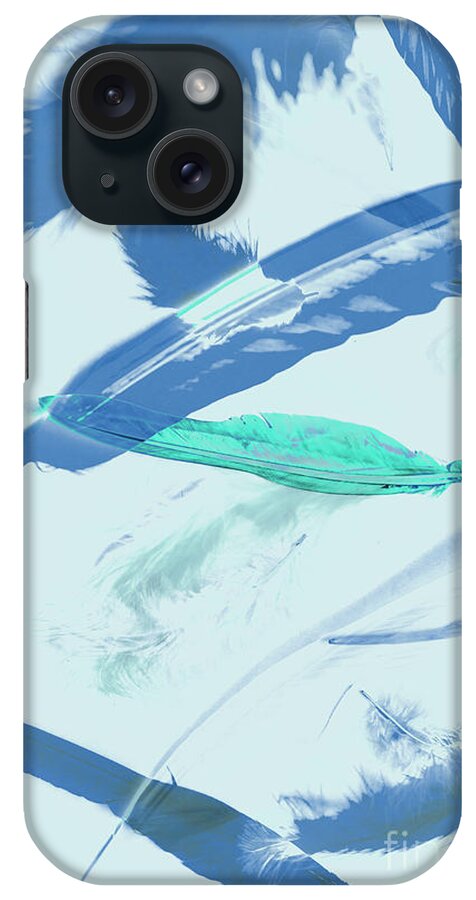The image depicts the back of a smartphone encased in a distinctive and vibrant phone cover. The phone’s dual camera lenses are prominently located in the top left corner, set against a black surround that contrasts the main color scheme. The cover itself features an abstract design on a white background reminiscent of snow, with a dynamic interplay of feather-like or brushstroke patterns in varying shades of blue and turquoise. These shapes, appearing as splashes or streaks, form X or V shapes across the surface, lending a sense of movement and artistic flair. In the bottom right corner, there is a watermark or logo displaying the letters "F-I-L." The overall design is visually striking, combining elements of art and function to create an aesthetically pleasing look for the smartphone.